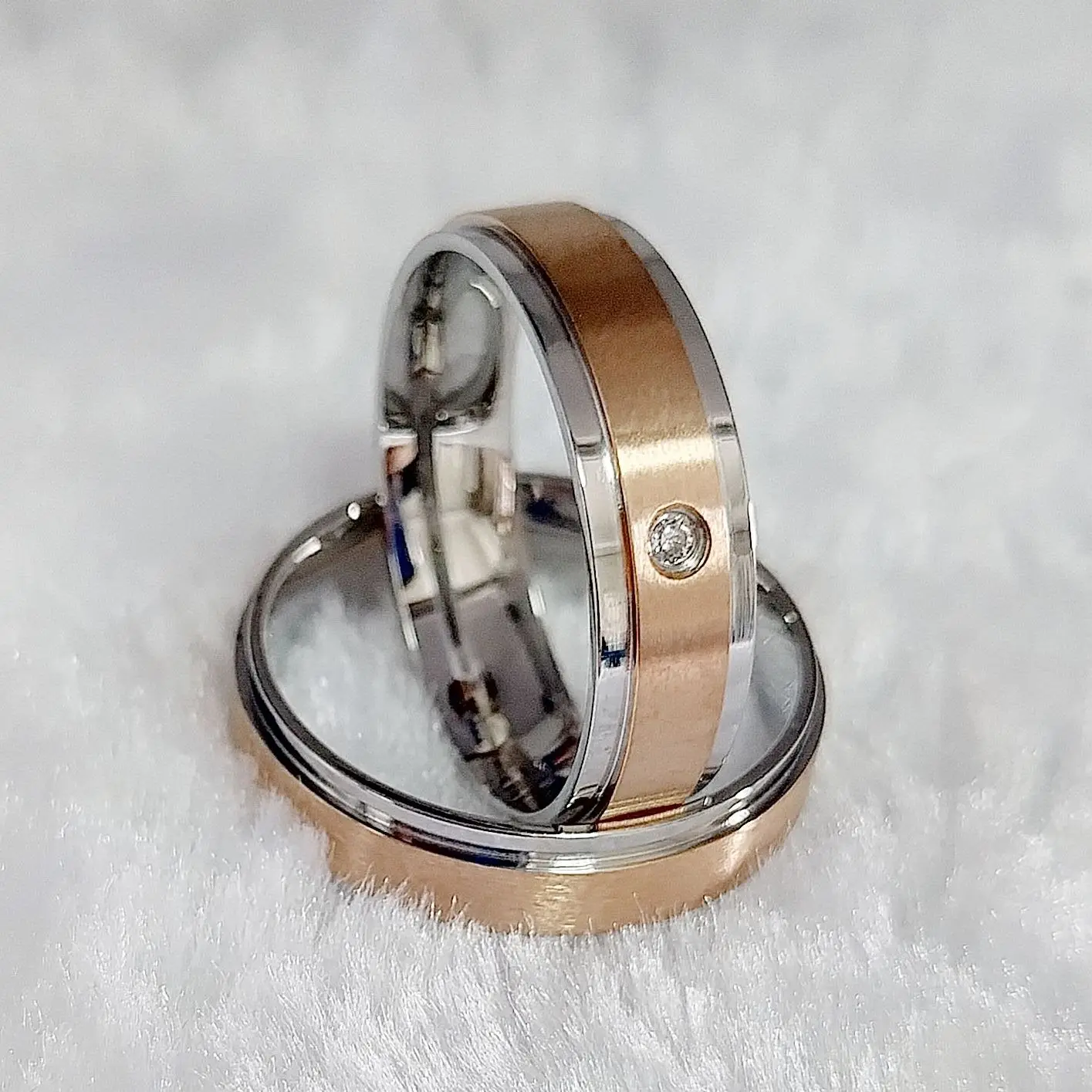This photograph captures two two-tone rings resting on a soft, furry white surface. Each ring features a distinctive design, with a silver outer band and a smaller band of rose gold running through the center. The focal point of both rings is a single diamond, set slightly within the band rather than flush on top, adding a layer of depth and intrigue. One ring is laid flat, while the other stands upright inside the first, angled slightly to the right. The rings reflect light beautifully, highlighting their shiny metal interiors and creating subtle reflections. The image predominantly showcases the contrast between the silver and rose gold tones, with a hint of white and black in the mix. The backdrop's texture emphasizes the rings’ elegance, making it unclear if the photo was taken indoors or outdoors, but the emphasis is clearly on the luxurious and intricate details of the rings themselves.